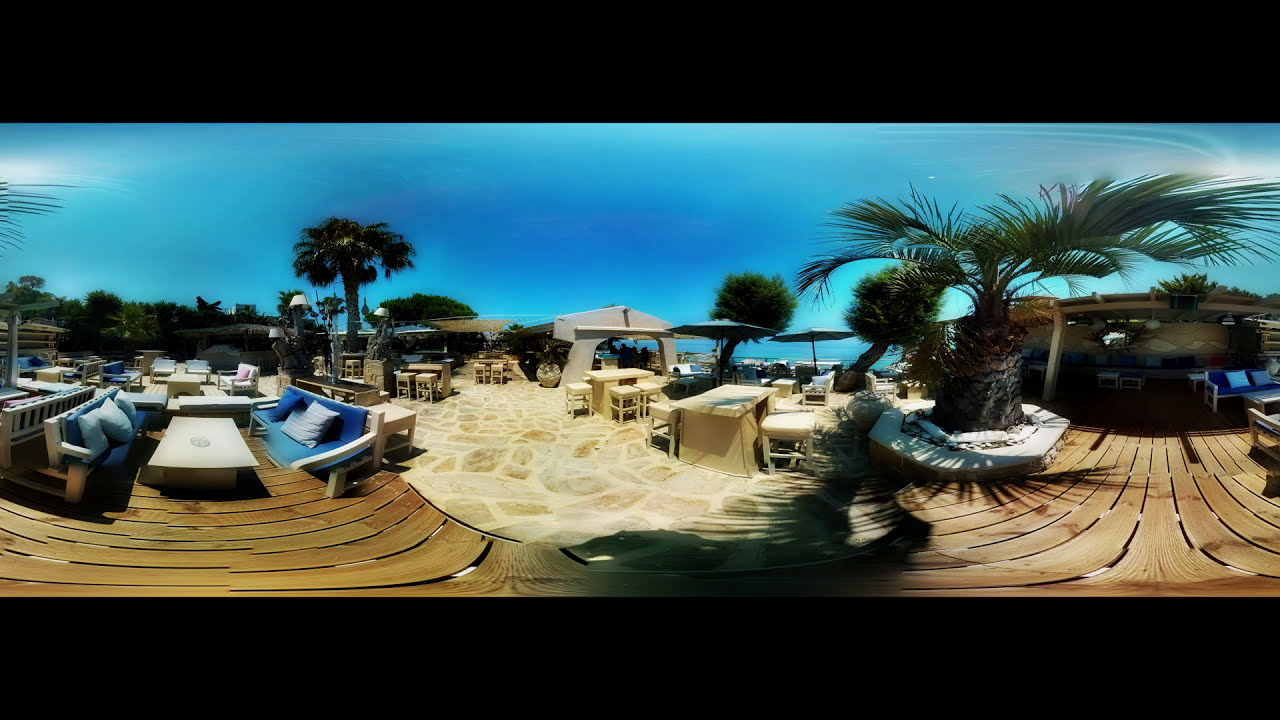This panoramic photo of a tropical resort captures a serene beachfront deck adorned with furniture and lush greenery under a clear blue sky. The image, likely taken from a beach camera, features a wooden deck stretching across the foreground, populated with white tables and blue-cushioned seating. On the left side, a white table is flanked by benches adorned with blue cushions and white pillows, resting on the light brown, tan-colored wooden floor. In the center and extending to the background, additional tables and chairs are visible, interspersed with palm trees and regular trees, casting a tranquil and inviting atmosphere.

A distinctive feature on the right side includes a large sago palm situated in an octagon-shaped concrete planter, surrounded by more seating with matching blue cushions. This decked area on the right continues under a large awning, which might be a bar area, providing shade and enhancing the resort’s relaxing ambiance. The perspective of the photo presents a slight curvature, adding to its unique visual appeal. The scene, devoid of people, is bathed in bright sunlight, illuminating the entire setting and highlighting the resort’s luxurious and tranquil atmosphere.